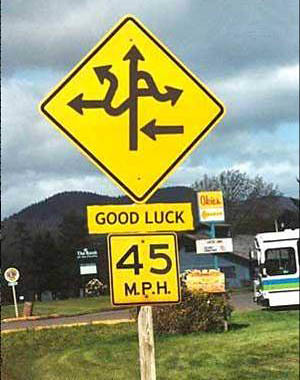The image is a vibrant color photograph capturing a street sign in a mountainous or hilly region. Dominating the top half of the image is a clear sky, with rolling hills and several trees forming a serene background. In the middle ground, there's a prominent yellow diamond-shaped street sign affixed to a vertical pole. This sign features a black arrow pointing straight ahead, accompanied by two additional black arrows beneath it, both pointing to the left. Below these arrows, there's a smaller horizontal yellow sign displaying "Good Luck" in bold black letters. Beneath this, another yellow square sign with a black border shows a speed limit of "45 MPH" in black text.

In the background to the right, part of a bus is visible, adding a touch of urban life to the rural scene. The foreground features a small patch of grass in the lower left-hand corner. A narrow street is lined with tree trunks, guiding the eye through the image. Additional signs are present: one with the Lions Club logo, another vaguely advertising an unknown entity, and a third presumably for a restaurant, characterized by its white and yellow coloring but devoid of any distinguishing text.